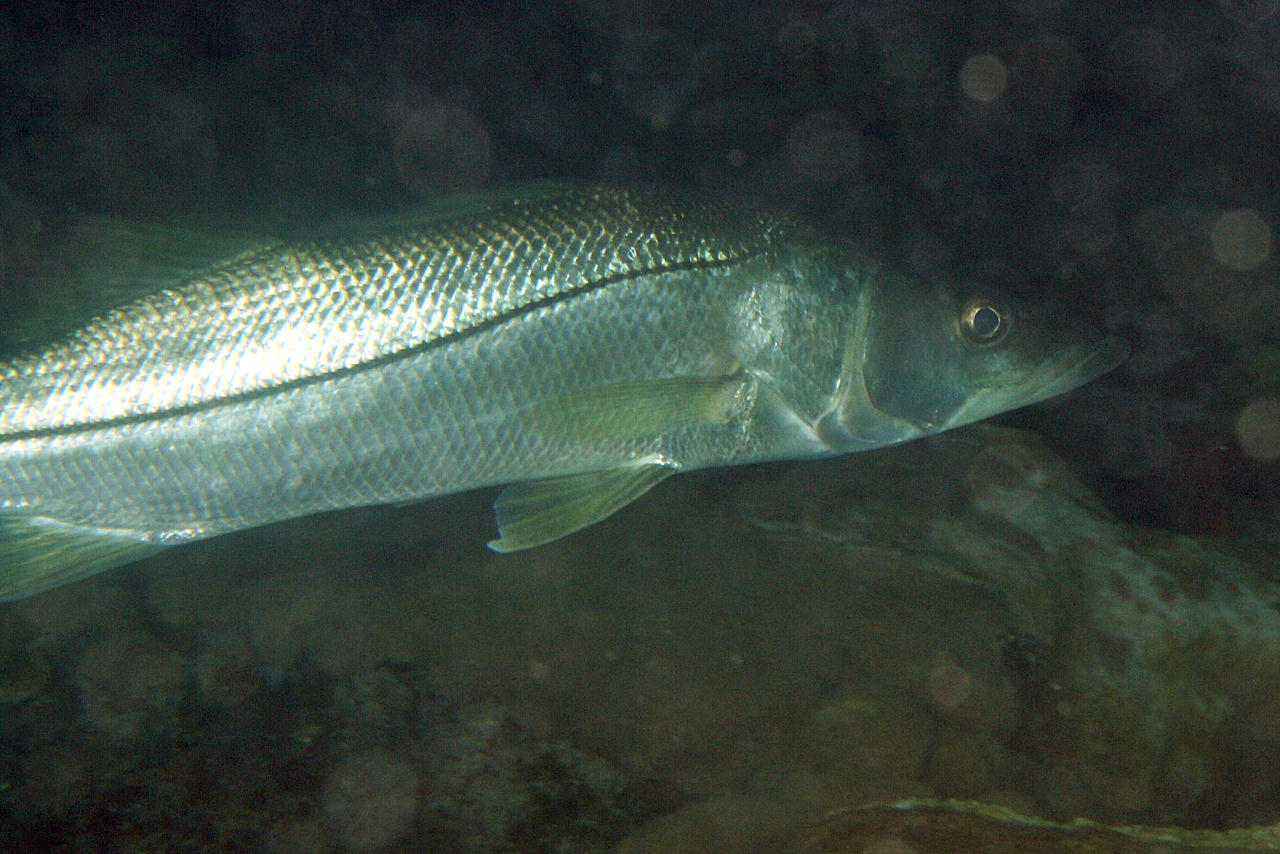This is a close-up photograph of a long, shiny fish, predominantly greenish with an iridescent, silver, and somewhat scaly appearance. The fish resembles a barracuda and is captured while swimming in water. It is facing and moving to the right side of the frame, displaying its right eye—a golden eye with a black circle in the middle. The fish has a thin, triangular face and small, slightly yellow-tinted fins. A distinct line runs down the side of its body. Light reflects off the fish's scales, creating a shimmering effect. The background consists of dark green, black, and brown rocks, some covered in algae, contributing to the impression of a natural, though somewhat murky, aquatic habitat. Light bubbles can also be seen, enhancing the texture and depth of the image.